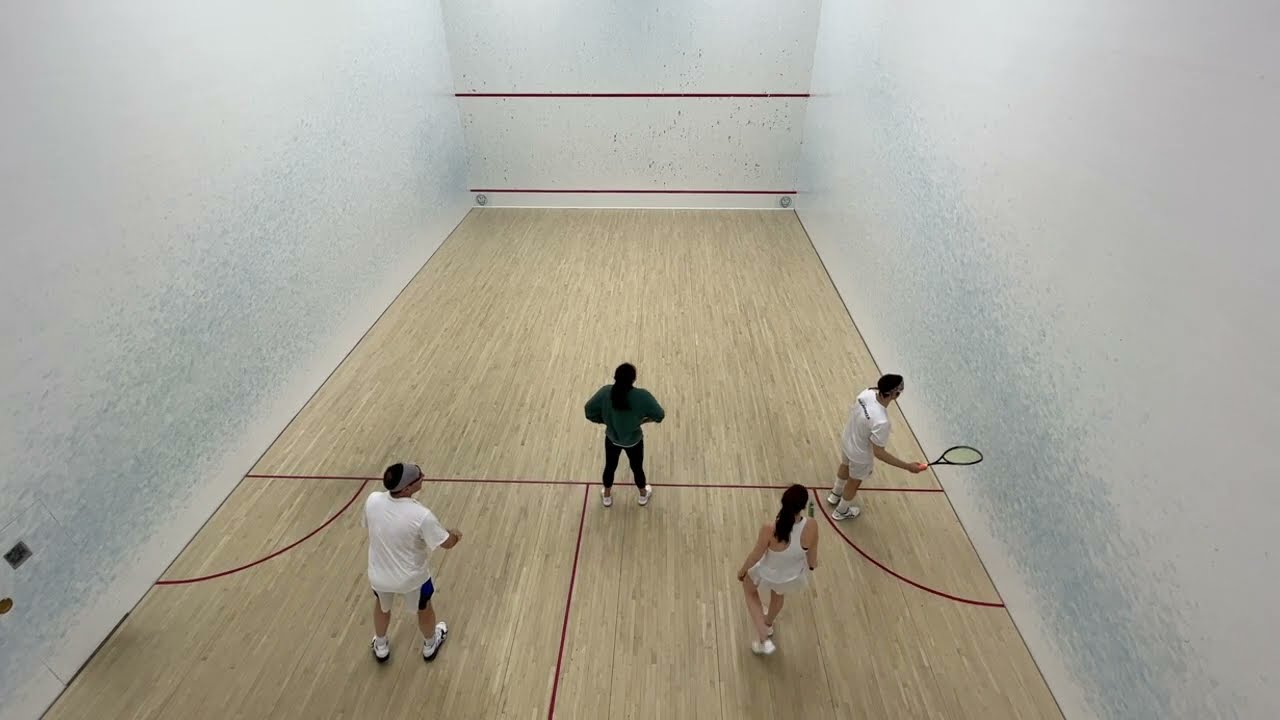The color photograph captures an indoor racquetball court viewed from an elevated vantage point, either by a drone or an observation platform within the room. The court features three white-painted walls, with chipped paint at the bottom revealing a light bluish hue. Two red pinstripes adorn the far wall. The floor is made of light brown wood, marked with a horizontal and a vertical red line bisecting the center, complemented by two beveled red lines on either side.

Four people are positioned on the court, all facing away from the viewer. In the center near the horizontal red line stands a person in a black long-sleeve top, black pants, and white shoes, posed with arms on their hips. To the left, a man in a white short-sleeve shirt, white pants, and white shoes wears a visor and is facing to the right. Below him and slightly to the left, a woman with long dark hair, dressed in a white tank top and white skirt, is positioned. On the far right stands another man in a white shirt and shorts, holding a racquet in his right hand. The carefully framed image captures the quiet anticipation of the players in a realistic and detailed manner.